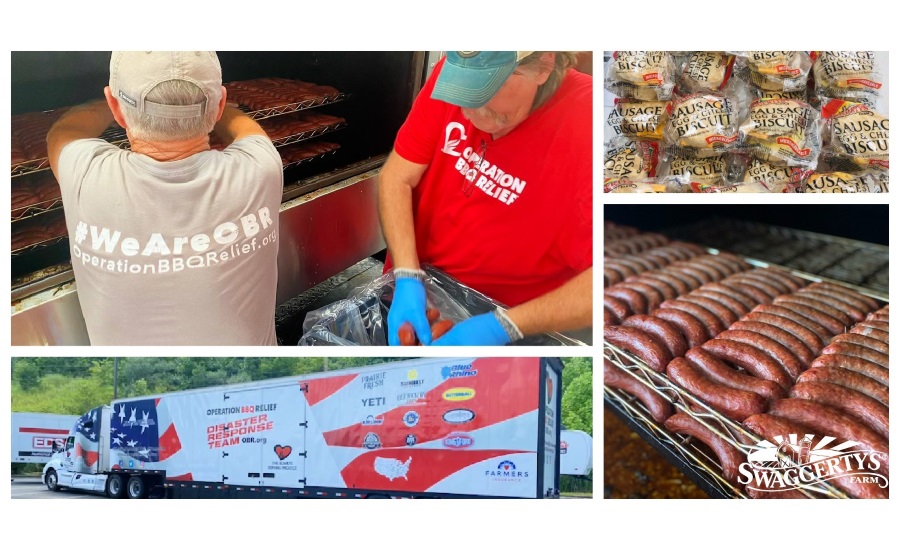This image is a detailed collage composed of four distinct yet related photographs, all centered around the theme of sausage preparation and disaster relief. In the top left, the largest photograph captures an activity scene with two individuals engaged in the process of making sausages. The person on the right, a woman wearing a red shirt emblazoned with "Operation BBQ Relief" and blue gloves, handles sausages with careful attention. To her left stands a man whose back is turned, revealing a gray shirt that reads "We Are OBR Operation BBQ Relief dot org." He appears to be placing sausages into an oven or similar cooking apparatus, contributing to the collective effort.

Directly below this primary image, there's a vibrant photograph of an 18-wheeler semi-truck, prominently decorated with American flag motifs and inscribed with “Disaster Response Team,” emphasizing the mobilized community support. To the left of this truck image are two smaller, vertically-aligned photographs. The top one is a close-up of sausage biscuits, individually wrapped in packaging that clearly labels them "Sausage Biscuit." Beneath it, the final photograph showcases a neat row of fully cooked sausages, ready for consumption. This imagery encapsulates not only the preparation process but also highlights the variety of food items and the logistical support involved in the relief efforts.